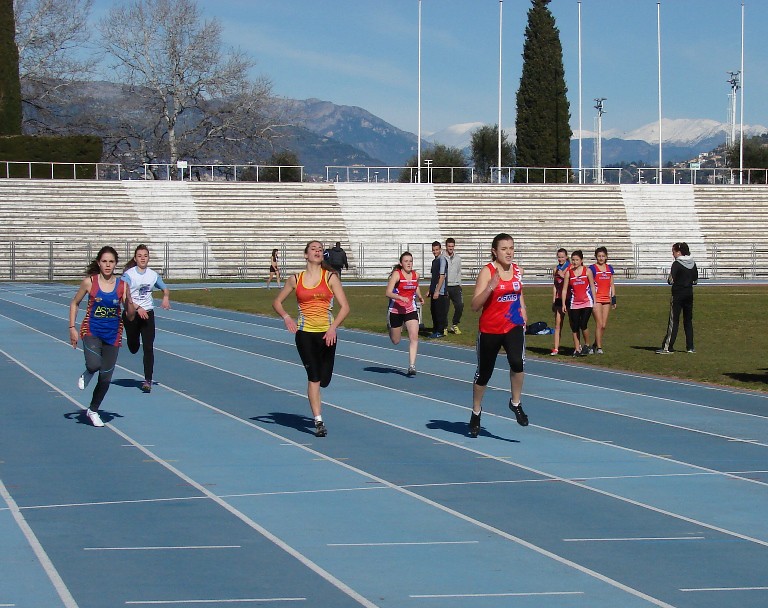This rectangular photograph captures a lively scene on a university or high school running track set against the stunning backdrop of a mountain range and a bright blue sky. The track itself features alternating dark and light blue lanes with white lines dividing each lane. In the foreground, several young girls are mid-run, some wearing red track tops with black bottoms, while others sport unique outfits such as an orange top with black bottoms, a white and blue top with black bottoms, and a blue and red top with gray bottoms. The activity could be a race or a training session. 

In the middle of the track and nearby grassy area, a mix of figures can be seen: additional girls standing around, possibly taking a break or awaiting their turn, a coach dressed in a jacket and pants who stands taller than the rest, and a pair of gentlemen in the background. Surrounding the track are empty bleachers, indicating the absence of spectators and suggesting this is likely a training exercise rather than a formal event. The serene mountain range and scattered trees in the distance enhance the picturesque quality of the scene.